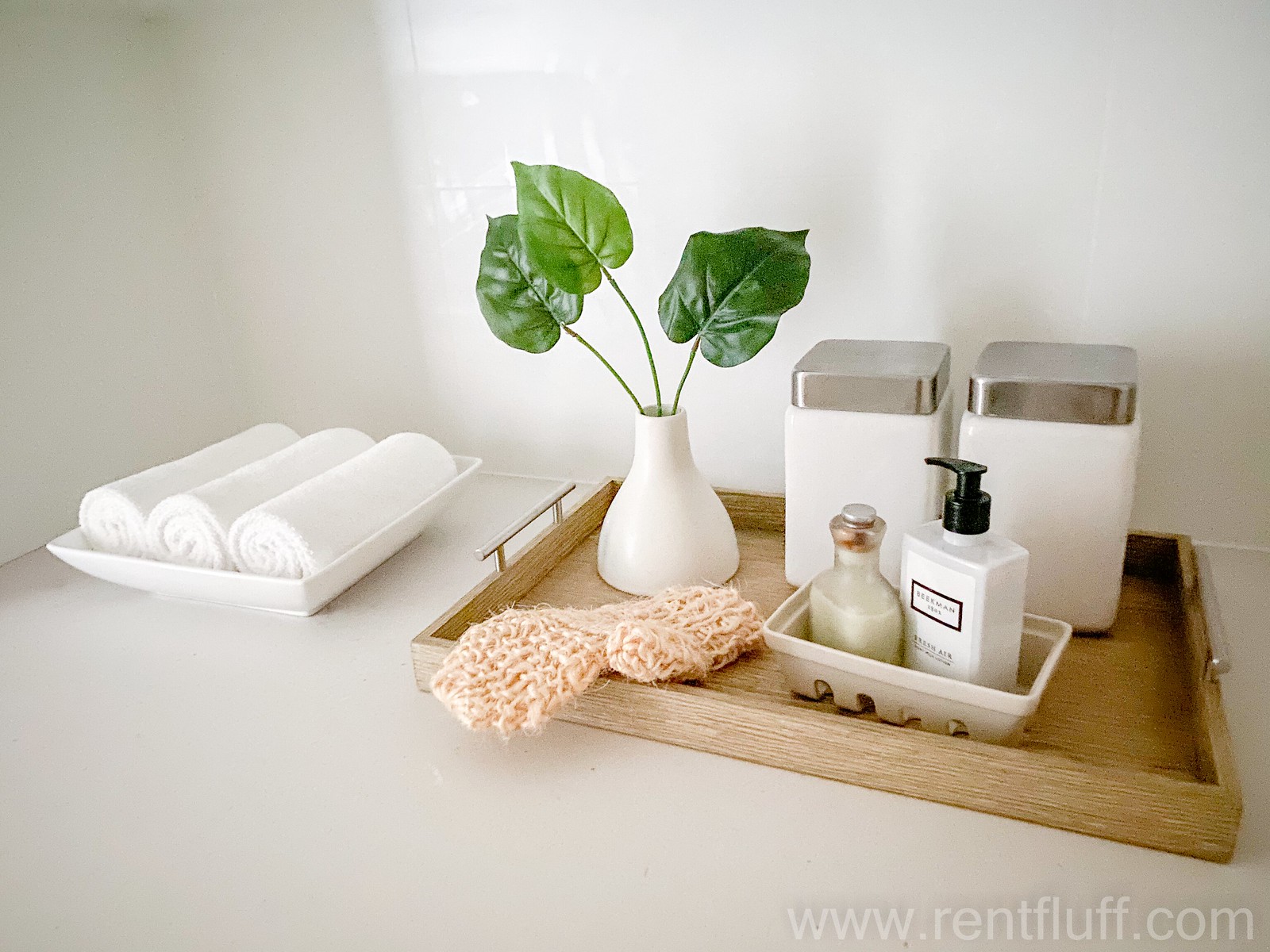The image resembles an advertisement for a luxurious home spa setup. Centered in the composition is a pristine white rectangular saucer, slightly angled to the left, containing three neatly rolled white towels. Behind this saucer is a white wall that starts midway on the left side and angles upward, then disappears behind the saucer before re-emerging and angling downward to the right, continuing behind a finely crafted brown wooden tray. The tray, extending nearly to the right edge of the frame, is angled downward and features elegant silver-gold handles on each end, supported by small bars.

In the top left corner of the tray, a sleek white vase with a flared base and a tapered neck holds two green leaves, one slightly overlapping the other, with another leaf extending to the right. Resting gently over the bottom edge of the tray is a delicate knitted glove, slightly hanging off toward the left. To the right of the vase, two white rectangular jars with square silver lids stand side by side. In front of these jars, a small white dish is angled slightly to the left, and next to this, a tiny glass container with a silver top.

Adjacent to the glass jar, there's a square-shaped soap dispenser with a black pump pointing to the left. The entire setup is showcased on a white table, against a pristine white backdrop, exuding a serene and sophisticated ambiance. In the bottom right corner of the composition, the URL www.rentfluff.com is subtly inscribed in light white lettering, completing the elegant presentation.